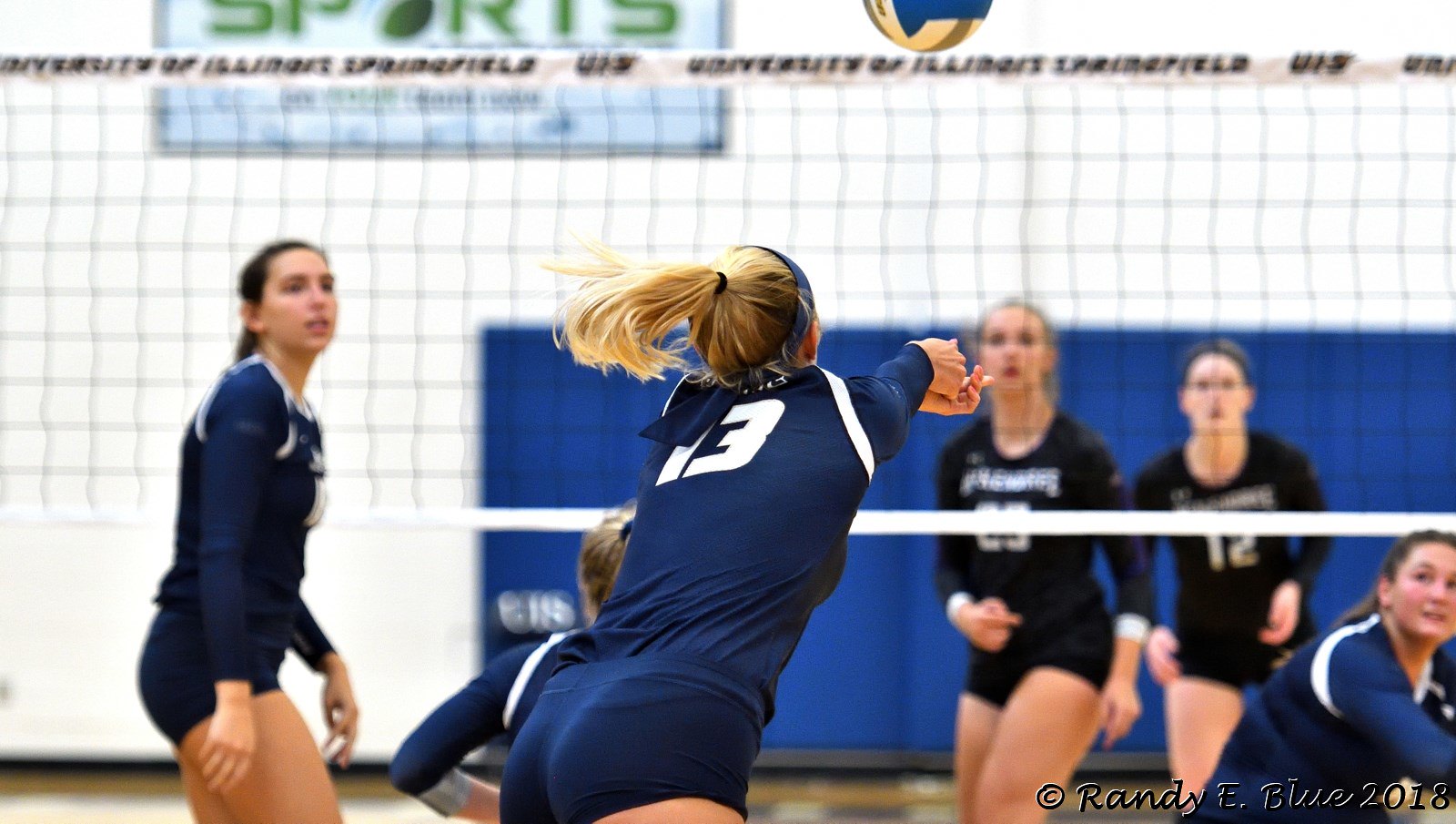This photograph captures an intense moment in an indoor girls' volleyball match. The scene is set on what appears to be a hardwood floor, defined by a prominent white volleyball net stretched across the center. On one side of the net, we see a player from the team dressed in blue uniforms diving forward with outstretched arms, her focus on the volleyball descending towards her. This player, identifiable by her number 13 jersey and blonde ponytail, is captured mid-action, appearing to fall away from us. Flanking her are two teammates; one, partially visible and on the ground, and another to the left with brown hair in a ponytail, watching the ball intently.

On the opposite side of the net, three players in black uniforms are positioned. One girl has the partially obscured number 29 on her jersey, while the girl next to her displays the number 12. Another player on their team is seen on the ground, also fixated on the ball. The background includes a white wall with a large blue rectangular mat or padding, and a blurry white sign with green print reading "sports". On the bottom right of the image, small text reads "© Randy E. Blow 2018," indicating the photo's copyright details. The ball is visible near the top of the image as everyone converges, underlining the fast-paced action of the match.